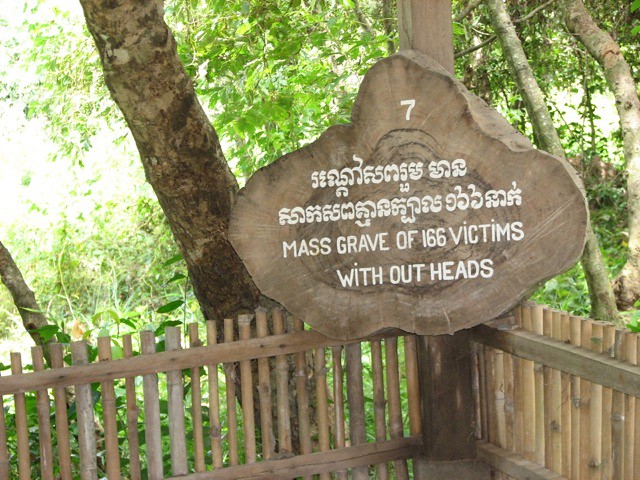This photograph features a somber outdoor placard crafted from a tree stump cut into a log. The log is affixed to a wooden fence positioned against a lush, dense forest, suggesting it might be located in Southeast Asia. The sun highlights the vibrant green leaves and plants in the background. The placard prominently displays the number "7" in white at the top. Beneath this, there is text in what appears to be a Hindu or Middle Eastern script, followed by its English translation: "Mass grave of 166 victims without heads." The photograph captures the poignant memorial with a flash, causing a reflection off the wooden or bamboo fence that supports the log. The setting appears to be a museum or a commemorative site porch, adding an element of reverence to the depicted scene.